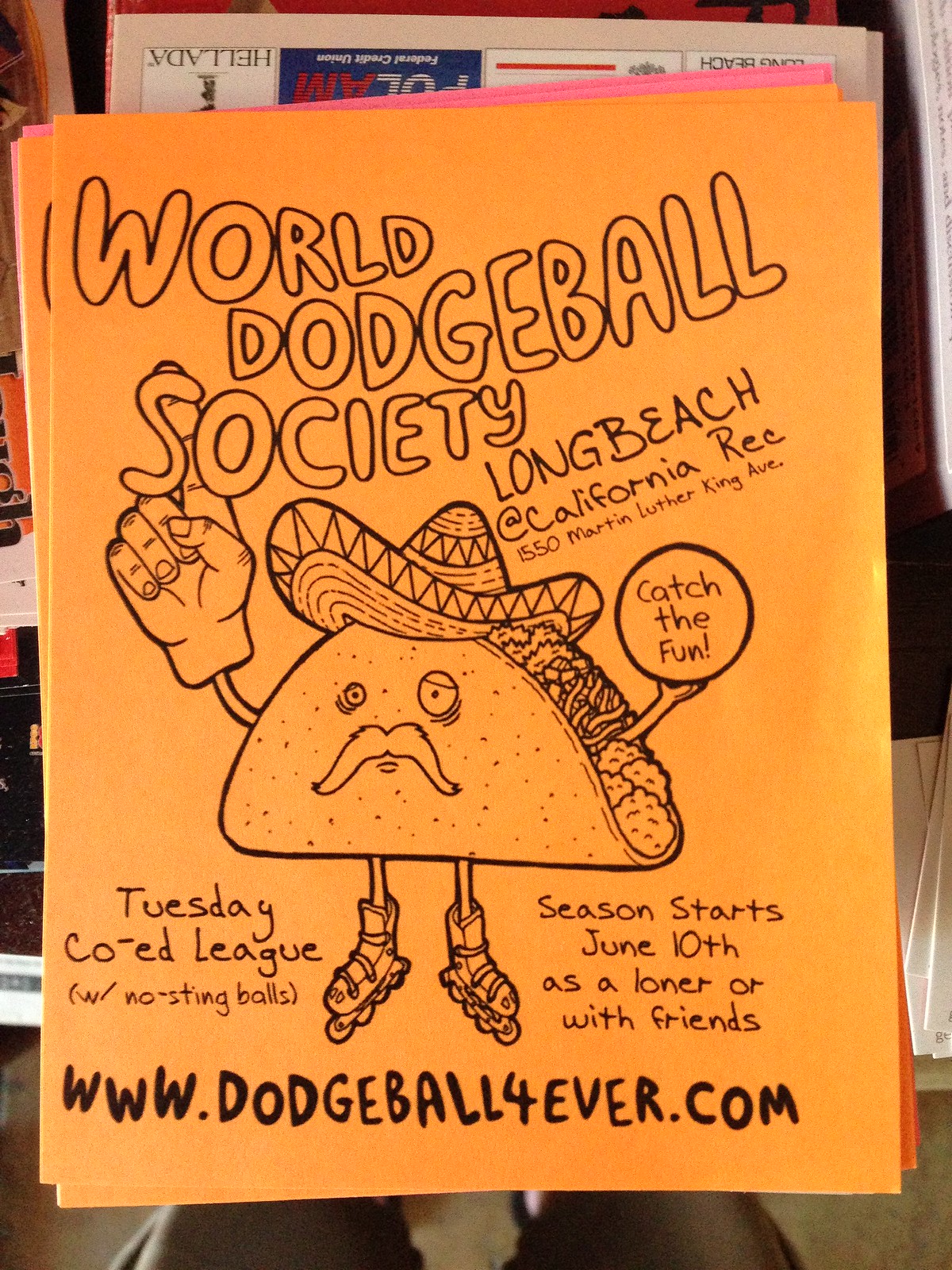The image showcases an advertisement on an orange flyer for the World Dodgeball Society, Long Beach at California Rec, located at 1550 Martin Luther King Avenue. The advertisement, designed in a playful and artistic style with bubble letters, features a whimsical illustration of a taco with a human face. The taco character is adorned with a sombrero, a large bandito mustache, and is wearing rollerblades. Adding to its quirky charm, the taco holds a circular sign that says "Catch the Fun" and sports a monocle-like swollen eye. The flyer promotes a co-ed dodgeball league starting on June 10th, inviting participants to join as a loner or with friends. Essential details like the website dodgeballforever.com (with '4' as the number) are also included. This fun and creative flyer captures attention with its unique and positive design.